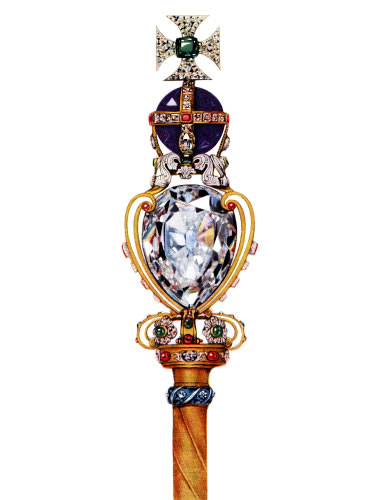The image showcases a highly ornate, slender staff set against a stark white background, positioned centrally to highlight its intricate details. The staff is richly adorned with various gems and intricate designs, creating an impression of regality and craftsmanship. At the very top, the staff features a stylized Maltese cross, embellished with a green gem at its center. Below this cross is a circular purple gem, intersected by another cross-like design formed by smaller gems and diamonds. The middle section of the staff boasts an imperial diamond-shaped gem with a sharp arrowhead base, flanked by gold flourishes. Further down, a crown-like ornamentation adds to its majestic appeal. The staff is primarily gold in color, with silver clasps and a heart-shaped golden detail. The wooden handle at the bottom ends in a swirl design, accented with two red gems and encircled by a blue ring. The overall color palette includes vibrant shades of yellow, green, purple, red, blue, and gold, making it a visually captivating object, possibly depicted in a stock image or a novelty wand advertisement.